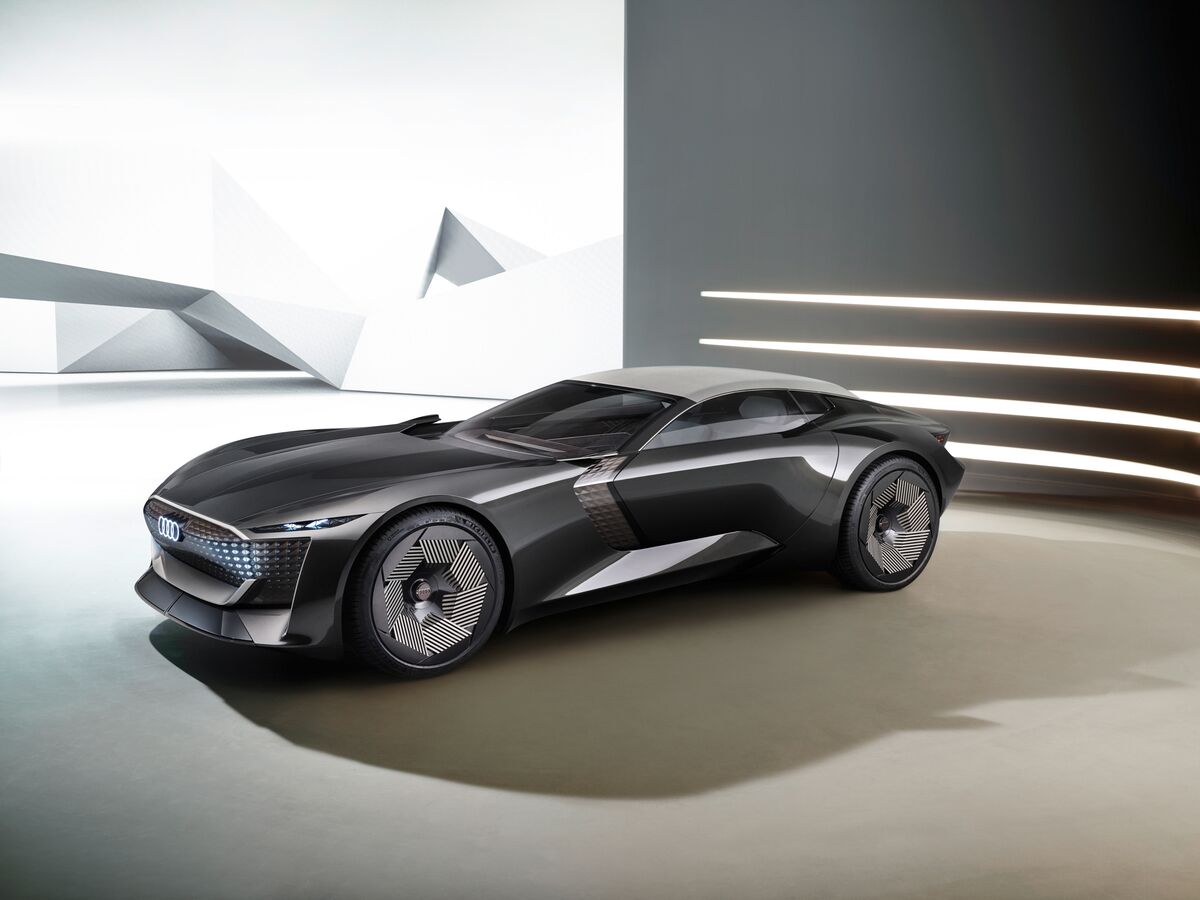The image showcases a computer-generated, futuristic concept sports car, likely made by Audi. The sleek, muscular vehicle is predominantly black, exuding a fast and aggressive aesthetic with narrow, angry-looking front lights. The car's wheels feature intricate designs with carbon fiber looks, black and silver interspersed across the rims, and the inner bars forming geometric patterns that would create a mesmerizing effect when spinning. 

Displayed from a side view, the car is set against a split background: the upper left is a light grayish-white adorned with geometric shapes, while the right half is a dark gray-black, featuring white stripes at the bottom. The car casts a large shadow on the white ground beneath, emphasizing its form. The silver and black stripping along the side and the accentuating silver bumper and emblem further enhance its modern appeal. A subtle yet striking addition is the thin white line above the front grill, contributing to its advanced design.